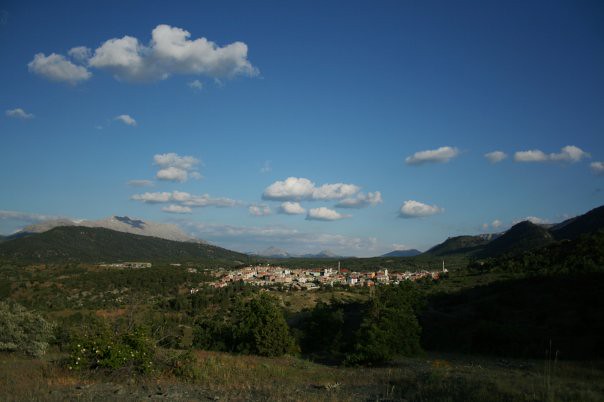The image presents a breathtaking vista dominated by a deep blue sky that transitions from a darker hue at the top to a lighter shade near the horizon. This sky occupies the upper 60% of the vertically elongated frame, peppered with sporadic white, puffy clouds. Below the sky, a series of rolling, dark green hills covered in lush foliage creates a dramatic scene. Nestled within these hills, the faint outline of a city comes into view, centralized in the lower portion of the image. The city's buildings appear small and primarily brown, suggestive of a European style, although this might be an artistic choice by the photographer rather than a true geographical indication. The cityscape, framed by the green slopes, includes various hues of brown and white, as well as some tall poles, possibly for power. At the front, small, non-substantial trees add an additional layer of depth to the lush, green panorama.